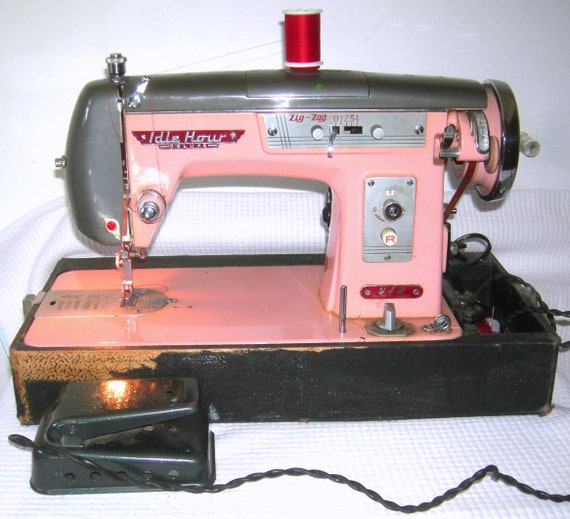The image is a color photograph in a square format, showcasing an antique, vintage sewing machine likely made by the company Eidel Hau. The sewing machine prominently features a retro aesthetic with a pink and gray color scheme. The body and riser portion are pink, with the gray areas primarily across the top and at the left front of the machine's head. The head faces left and the wheel, a pink metal with a stainless rim and handle, is on the right. Attached to the top of the machine is a bright red spool of thread. The machine also includes zigzag stitch capabilities, indicated by red lettering on a small metal plaque at the top left, which reads “zigzag.”

The sewing machine rests on a black base and has a black cord running across it and down to a foot pedal positioned in front on the left. It's set against an indoor background that is mainly white, with the surface it stands on covered by a blue and white checkered tablecloth. Light reflects off parts of the machine, particularly the clicking apparatus. The photograph combines elements of photographic realism with a distinctively retro and feminine ambiance.